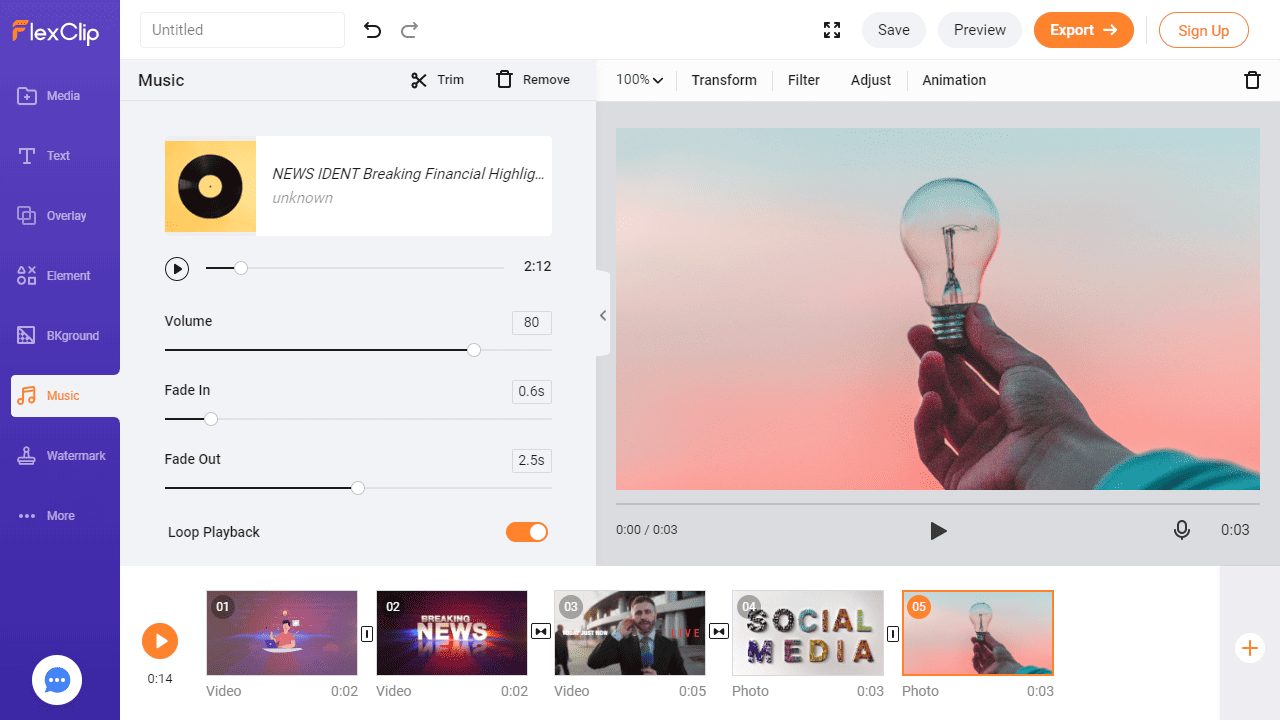Here is a detailed and cleaned-up caption for the described image:

"Screenshot of the FlexClip website user interface. On the left side, there's a blue, almost purple, sidebar with 'FlexClip' written in white, and the 'F' is highlighted in red. Below it, in gray text, are options listed as Media, Text, Overlay, Element, Background, Music (highlighted in orange on a white background), Watermark, and a 'More' icon represented by three dots. The top section is labeled 'Music,' with options for Trim, Remove, 100%, Transform, Filter, Adjust, and Animation.

The section also features various music categories such as News ID, ENT, Breaking, Financial, Hiding, Lighting, and Unknown. A play button is visible, showing a duration of 2 minutes and 12 seconds. The volume is set at 80%, with a fade-in time of 0.6 seconds and a fade-out time of 2.5 seconds. Loop-back functionality is enabled. The thumbnail image associated with the music shows a man's hand coming from the right side, holding a light bulb against a gradient background that transitions from peach at the bottom to light green at the top.

On the right side of the interface, there are buttons for Save, Preview, Export, and Sign Up. At the bottom of the screen, a series of video thumbnails are displayed, each lasting between 2 to 5 seconds, featuring various artistic visuals."

This formulation captures all the elements described and organizes them into a clear and detailed caption.